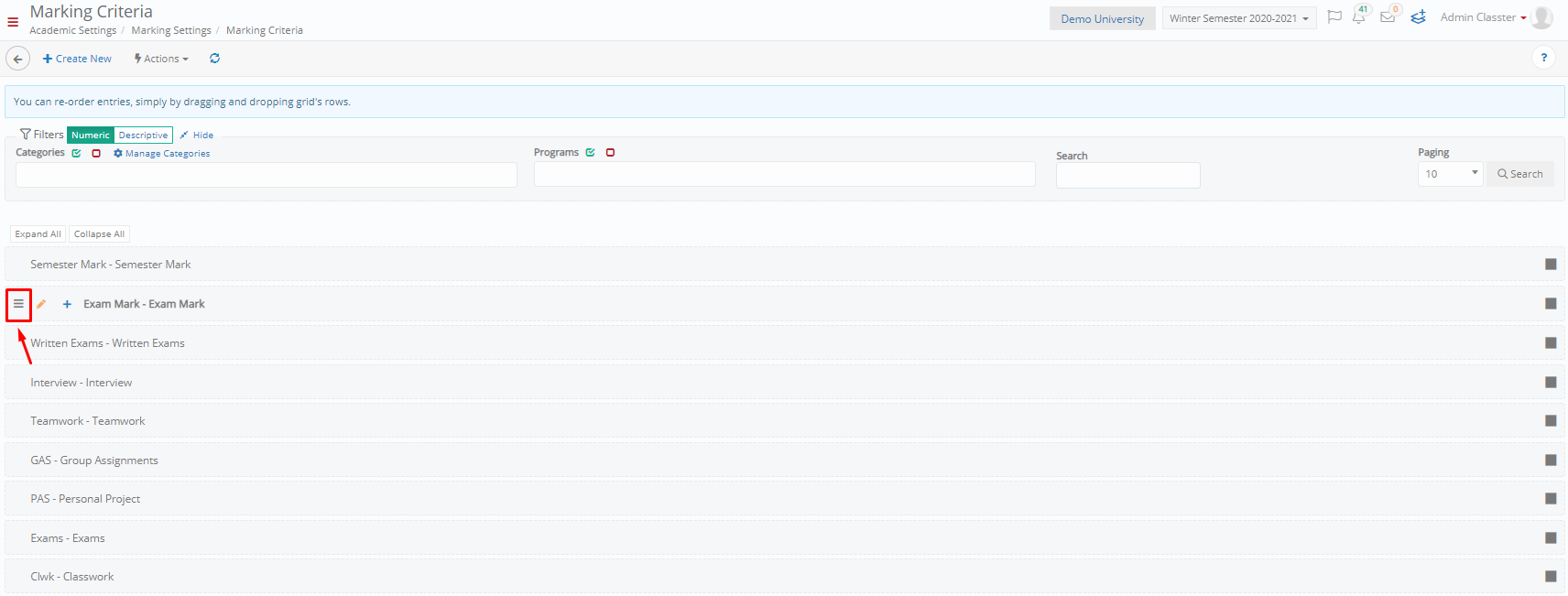The image appears to be a screenshot of a computer interface, set against a white background. The text within the image is small and blurry, making it challenging to read clearly. 

In the top left corner, the title "Marketing Criteria" is visible, followed by "Settings" and "Manage Settings" listed below it. The top right corner features various options, though their exact labels are unreadable due to the blur.

A gray section is present in the top portion of the interface, prominently featuring a blue button labeled "Create New" alongside an "Actions" menu. Below, there is a light blue section with dark, indistinct text.

Further down, there are input fields labeled "Categories" and "Programs," each accompanied by space for user input. A "Search" field and a corresponding search box follow these input areas.

At the bottom of the interface, multiple selectable options are arranged, with one option specifically highlighted by a red box and an arrow pointing to it. However, the contents of this highlighted section are also too small and blurry to discern.